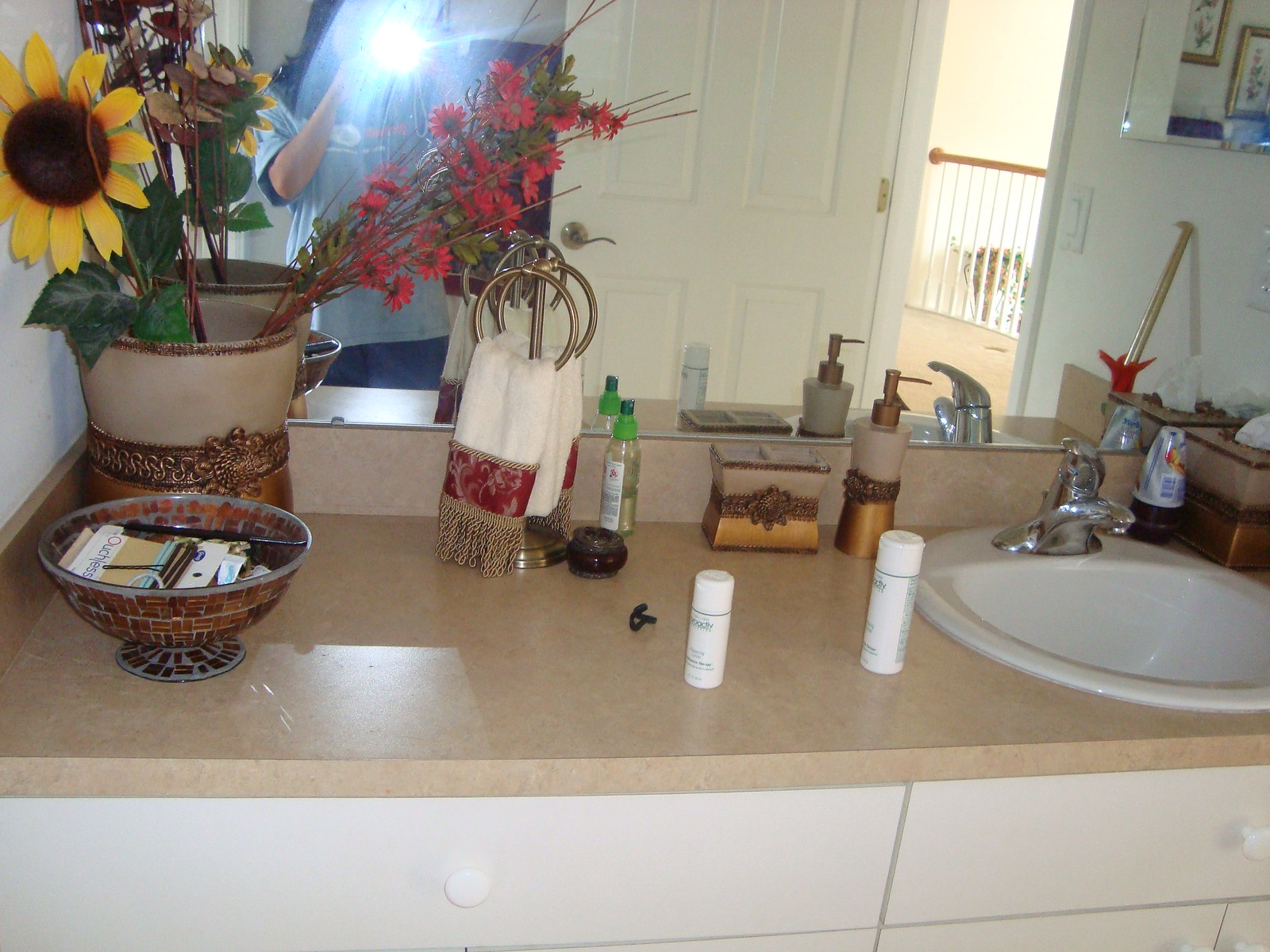This photograph showcases a well-organized bathroom countertop. The countertop itself is a beige color, providing a warm contrast to the stark white drawers below, which feature long handles with white plastic knobs. On the right side of the countertop, there's a pristine white, circular porcelain sink complemented by metal faucets.

Centrally positioned on the countertop are two cylindrical bottles of Proactiv, identifiable by their white packaging with green lettering. To the left of these bottles, a decorative brown vase adorned with bronze detailing stands out. The vase contains an arrangement of artificial flowers, including a prominent faux sunflower and vivid red blooms. In front of this vase, a sizable bowl is filled with hair accessories, including hair ties wrapped around a piece of paper packaging.

Adjacent to the vase and bowl is a bronze-colored towel holder, draped with a neatly folded white towel. Mounted on the back wall above the sink is a mirror, which captures the image of the photographer. Due to the flash, the photographer's face is obscured, but their attire is partially visible—a gray t-shirt and the top portion of blue bottoms. Reflected in the mirror is also a white door that leads to the rest of the house, adding depth to the scene.